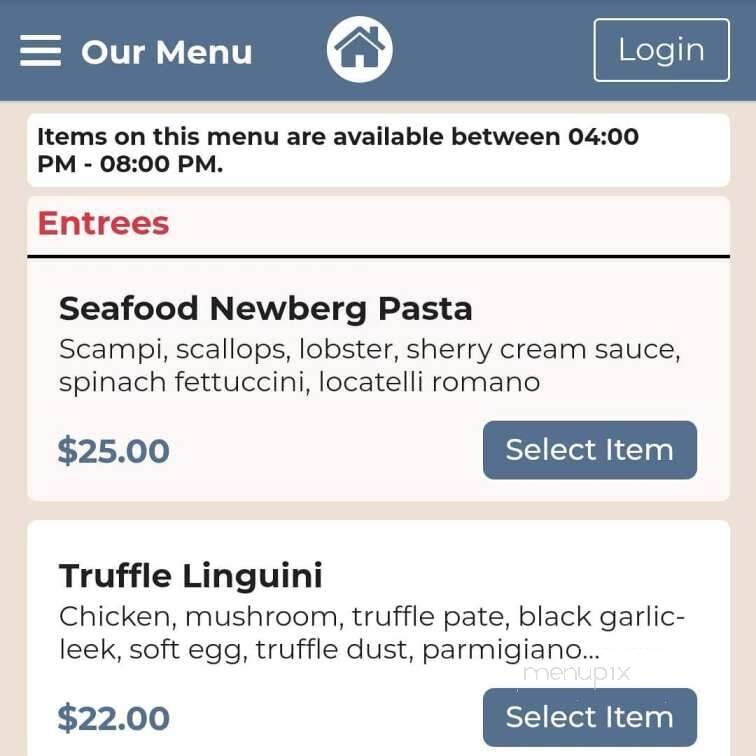At the top of the image, there is a thick header with a dull blue background. On the left side, three white lines indicate that clicking them will expand into a sub-menu. To the right of this icon is a bold, white, rounded sans-serif font displaying "Our Menu." In the center of the header, a white circular icon features a house illustration in the same bluish color as the background. Positioned on the right side of the header is a rectangular icon with a transparent background. This icon has a white rectangular border with rounded edges and contains the word "Login" in bold white letters.

Below the header, the background shifts to beige. A rectangular area with rounded corners and a white background contains bold black text. It reads, "Items on this menu are available between 04:00 PM - 08:00 PM."

Next, the background changes to a light peach color. At the top left of this section, the word "Entrees" is written in red, followed by a bold black line serving as a border. Below this, in bold black text, is the dish name "Seafood Newburgh Pasta." Beneath the dish name, in smaller non-bold lettering, are the ingredients: "Scampi, Scallops, Lobster, Sherry Cream Sauce, Spinach, Fettuccine, LOCATELLI Romano." 

Towards the bottom left of this section, there is a dull blue dollar sign followed by the bold price "25.00." On the right side, a rectangular icon with a blue background displays the text "Select Item" in white.